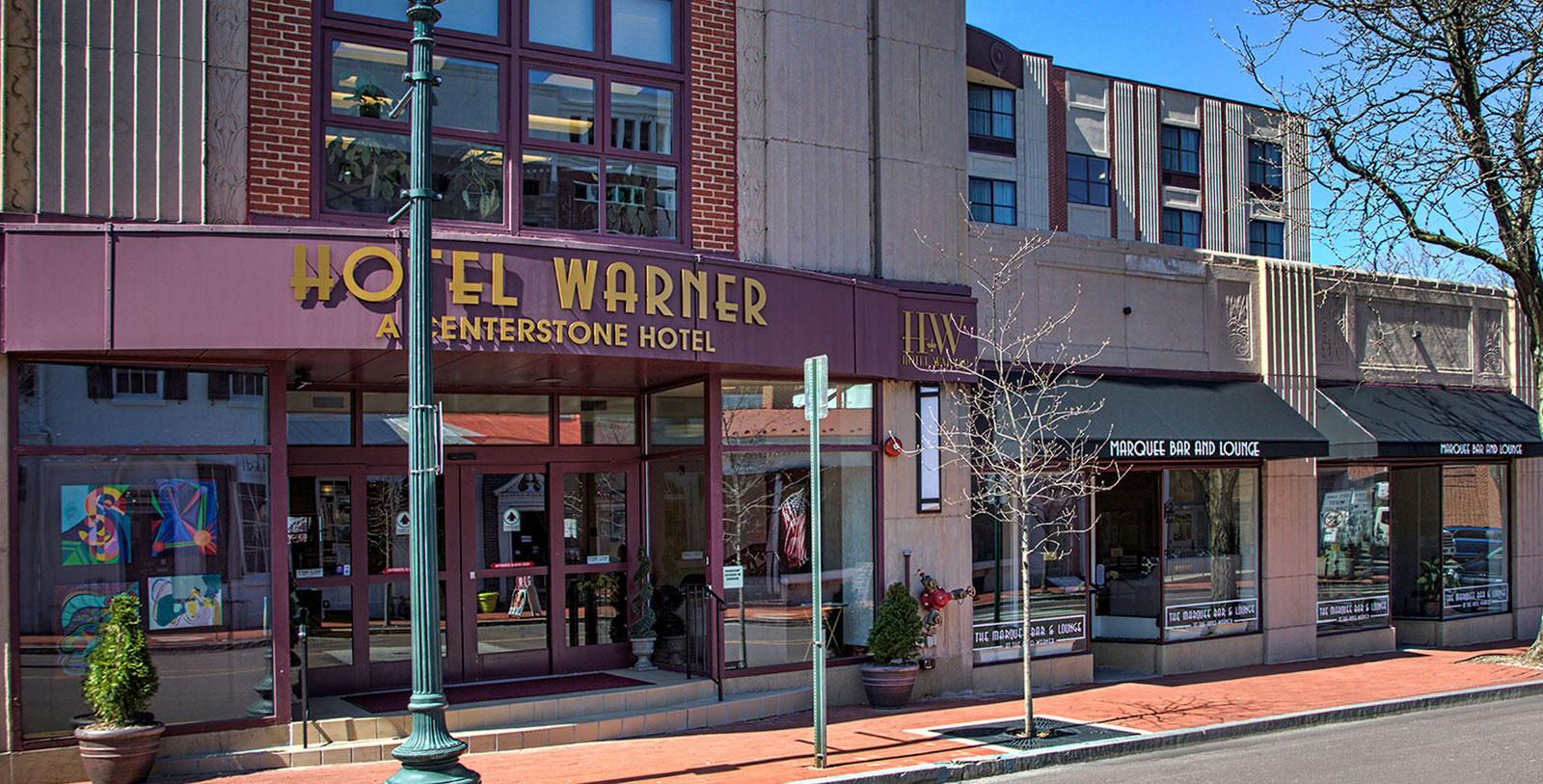The photograph captures a vibrant street scene on a clear day. Dominating the image is the multi-story Hotel Warner, a center stone hotel, with its striking reddish-purple arched facade prominently featuring its name in gold print. The hotel's double sliding doors and large windows are inviting, with potted plants flanking the entrance. Adjacent to the hotel is the Marquis Bar and Lounge, a smaller establishment that appears to be part of the same building but with separate entrances marked by identical signage. The bottom of the photograph shows a red brick sidewalk running alongside an asphalt street, adding texture and color contrast to the scene. A small tree grows in a designated area on the sidewalk, and a green street lamp and sign complement the urban setting. The upper right corner of the photo showcases a blue sky, adding a serene backdrop to the bustling street below.